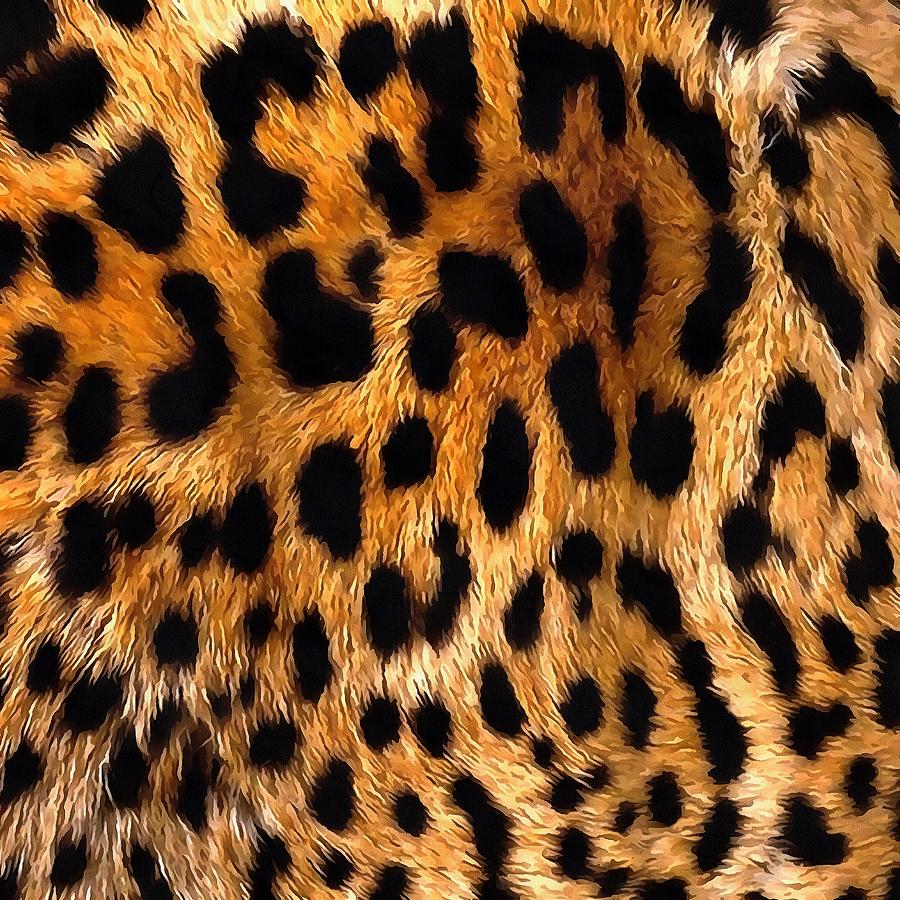The image appears to be an extremely detailed, close-up photograph of cheetah fur, capturing the intricate texture and color variations of the animal's coat. The fur is a rich orangish-tan color, adorned with a variety of black spots scattered unevenly across the surface. These spots vary widely in shape and size, with some resembling circles, ovals, or even irregular blobs. A few spots have distinctive shapes akin to a peanut or a candy cane. The photograph reveals individual hair strands, highlighting each one's unique curvature and the subtle shadows they cast. The fur color transitions from a darker tan at the top to a lighter, almost cream hue towards the bottom and right, reminiscent of the natural gradients in a cheetah's coat. This high-resolution image allows for a detailed view of the textures and the dynamic interplay of light and shadow across the fur.